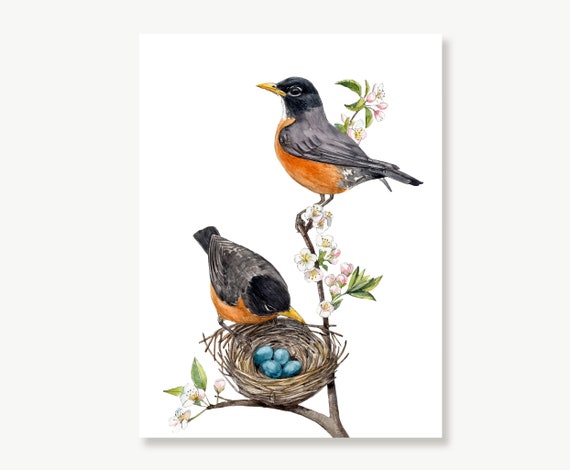This image is a detailed watercolor painting depicting two robins perched on thin tree branches adorned with green leaves, some white flowers, and small pink buds. One robin, characterized by its black upper body and orange-red underbelly, is perched towards the upper part of the image, looking left and keeping a vigilant watch. The second robin, similarly colored, is positioned in the lower left corner, peering down into a grayish-brown nest made entirely of twigs. The nest holds four bluish eggs. The overall color palette of the image includes white, green, pink, yellow, black, orange, brown, and blue, and the painting captures a calm and confident moment, suggesting the robins are likely co-parents overseeing their eggs.